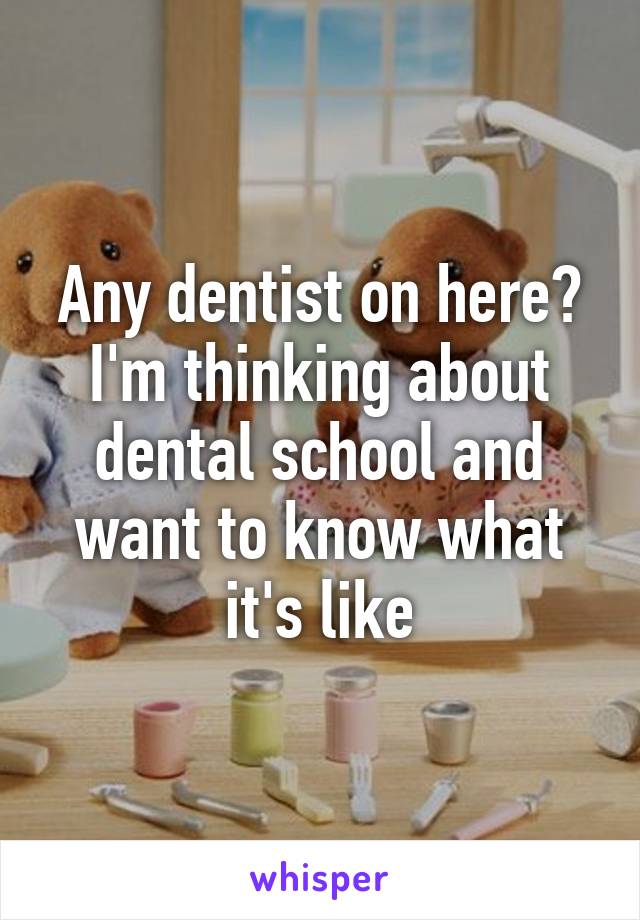The image features two stuffed animal figurines that resemble chipmunks or beavers, presented in a cartoon-like scene of a dentist's office. The figurine on the left, dressed in blue scrubs complete with a mask and holding a bag, appears to be a dentist. The figurine on the right, positioned in a dentist's chair and wearing a pink flower dress with a white bib, seems to be the patient. They both have human-like qualities, standing on two legs, and are looking directly at the camera. The background includes a window showing a bright blue partly cloudy sky, while the foreground displays an array of typical dental tools such as toothbrushes, various containers, and pastel-colored jars and cups. Overlaid on the image in white sans serif font is the text: "Any dentist on here? I'm thinking about dental school and want to know what it's like." The lower part of the image features Whisper's purple logo.